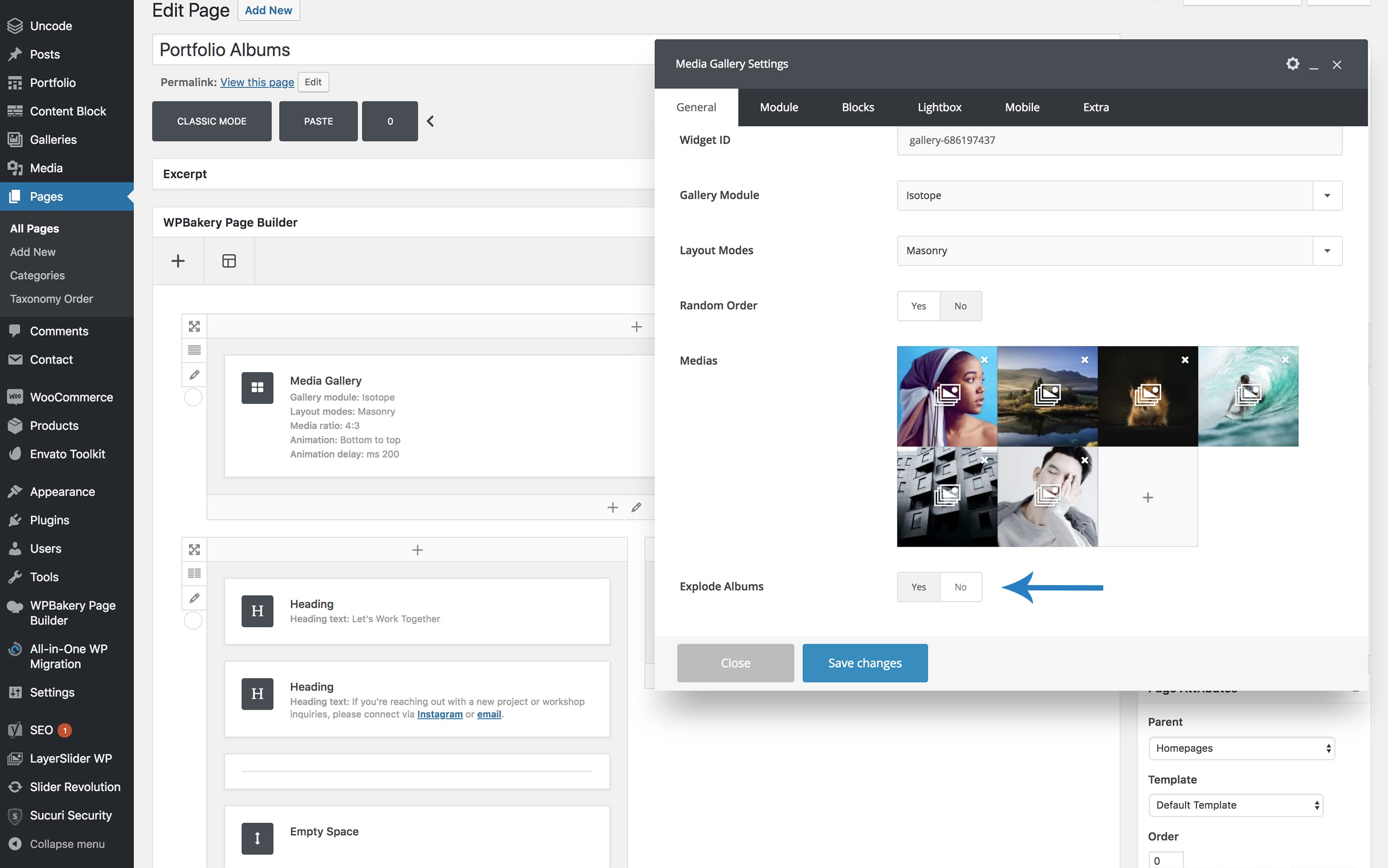This image is a detailed screenshot of a website builder interface, specifically from the Big Repage Builder platform. The screenshot prominently features a pop-up window overlaying the main workspace. 

The background workspace is a page editing interface labeled with sections such as "Portfolio," "Albums," "Classic Mode," and "Base." The main editing canvas appears blank with placeholders for headings and content blocks.

On the left-hand sidebar, there is a comprehensive menu listing the following items:
- Unicode
- Post
- Portfolio
- Content Block
- Galleries
- Media
- Pages (with sub-options "All Pages" and "Add New")
- Categories
- Comments
- World Commerce Products
- Appearance
- Plugins
- Users

The pop-up window, which is the focal point of the screenshot, includes tabs and settings options such as:
- Media
- Gallery Settings
- General Modules
- Blocks
- Lightbox
- Mobile
- Extra
- Widget ID
- Gallery Module
- Layout Modules
- Random Order
- Medias (displaying six different images)

A blue arrow within the pop-up points towards a section with options to "Yes" or "No" for "Explode Albums." The pop-up window also includes options to close it using a gray box or to save changes using a blue box.